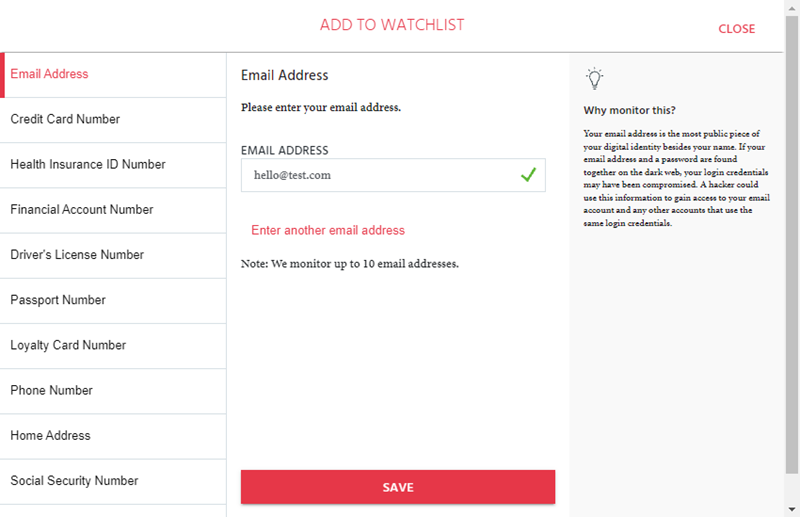**Detailed Caption:**

The screenshot depicts a webpage with a prominent interface for managing watchlists and personal information. At the top, the header features "ADD TO WATCHLIST" in large red capital letters, accompanied by the same text in smaller red capital letters to its right. Below this header, a horizontal gray line separates the main content of the webpage.

On the left side of the page, there is a vertical navigation menu. The top item on this menu, marked by a red vertical bar, is "Email Address" in black text. The subsequent items, listed in black with gray dividing lines between each, include "Credit Card Number," "Health Insurance ID Number," "Financial Account Number," "Driver's License Number," "Passport Number," "Loyalty Card Number," "Phone Number," "Home Address," and "Social Security Number."

In the central section of the page, the focus is on email address input. The text "Email Address" appears in bold black letters, followed by a prompt in smaller text: "Please enter your email address." Below this, another bold "Email Address" label is placed above a gray outlined input box containing the example email "hello@test.com." A green check mark is visible on the right side of this input box, signifying a correct entry, followed by a red warning message: "Enter another email address." Beneath this area, additional information is provided in black text: "Note: we monitor up to ten email addresses." At the bottom of this section, a red button with white text instructs users to "SAVE."

The right side of the webpage is grayed out, featuring a vertical informational box with a light bulb icon at the top. This section explains the importance of monitoring one's email address, stating: "Your email address is the most public piece of your digital identity besides your name. If your email address and a password are found together on the dark web, your login credentials may have been compromised. A hacker could use this information to gain access to your email account and any other accounts that use the same login credentials."

Finally, on the far right edge of the screen, a vertical scrollbar is visible, indicating the ability to navigate through the webpage's content.